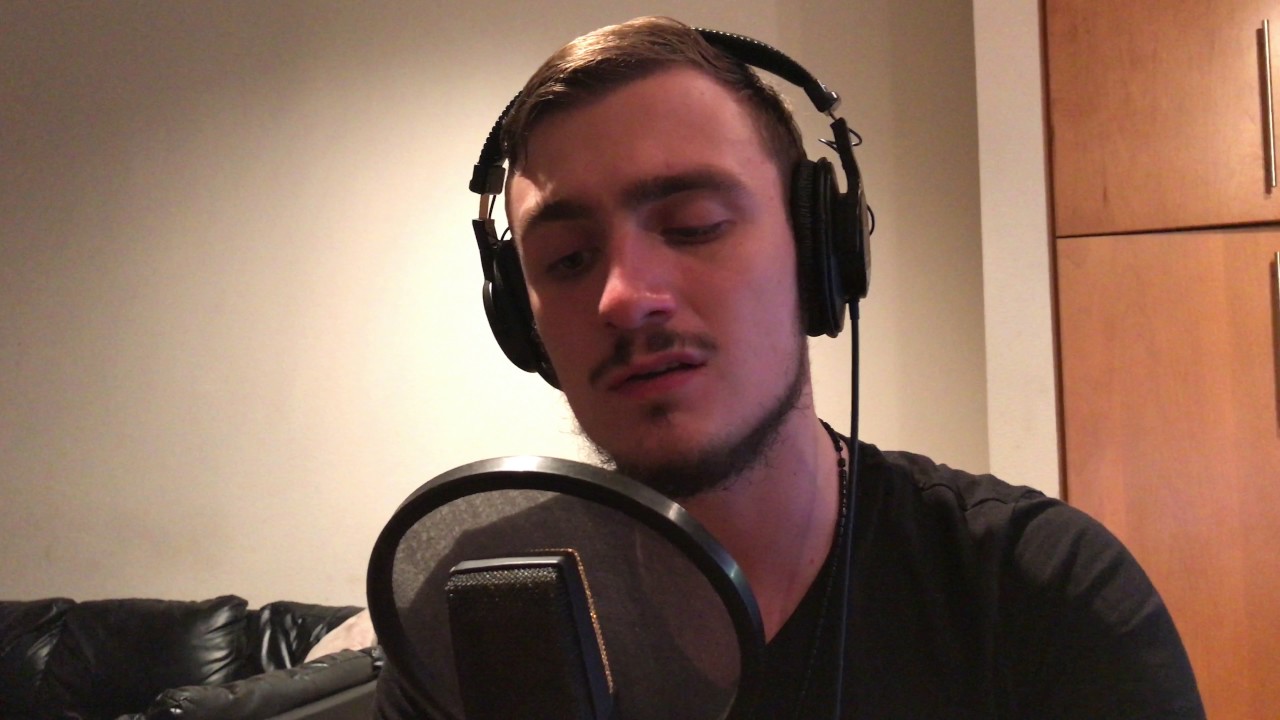A detailed photograph captures a man seated in a room, directly facing the camera. He is wearing black headphones and a black t-shirt, along with a black necklace-like accessory. His facial hair includes a mustache, a chin beard, and a neck beard. His eyes are half-closed, seemingly focused downward toward the black microphone positioned in front of him. The microphone is accompanied by a circular black pop filter. The background features a white wall; in the lower left corner, there is a dark, possibly leathery or pleather couch. On the right side of the image, a wooden cupboard with elongated metallic handles is visible.